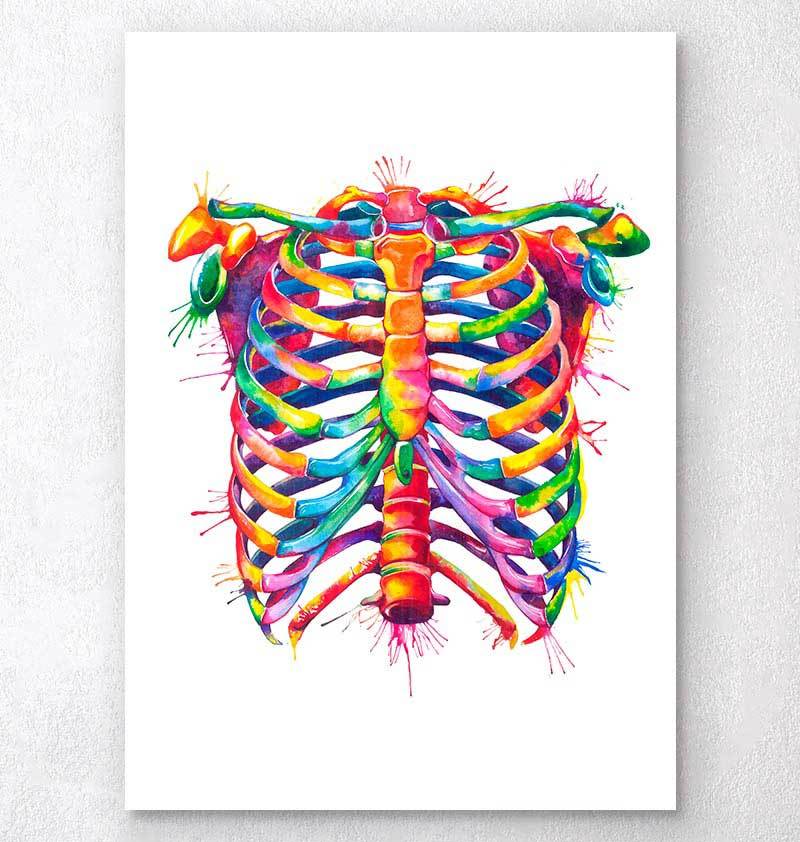The image depicts a vibrant, stylized painting of a human ribcage and spine, displayed vertically on a white background. The ribcage, positioned centrally within the artwork, showcases an array of rainbow colors including blues, greens, reds, oranges, and purples, creating a striking and lively composition. Each rib is multi-colored, contributing to the overall colorful aesthetic. The spine, running down the middle, is primarily adorned with shades of red and orange. Toward the top of the painting, the shoulder blades and sockets display hues of bluish-green and orange, enhancing the dynamic use of color. Additionally, there are three light, circular openings at the top corners of the ribcage, green on the left and blue on the right, adding an intriguing element to the detailed anatomy art.